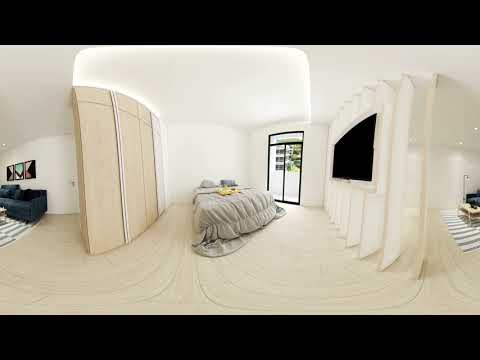The photograph is a horizontally aligned, rectangular image with thick black borders at the top and bottom. The setting is a bright, minimalist bedroom inside an apartment or house. At the center of the image is a neatly made bed dressed in gray bedding, which drapes onto the floor. Above the bed, there are sliding glass doors that open onto a balcony with a small white fence visible outside. The indoor flooring appears to be a swirled white tile, complementing the white painted walls.

To the left of the bed, there is a blue sofa positioned against a white wall adorned with three small pictures. A partial view of an adjacent room, likely a living room, is visible, where an area rug and possibly an end table can be seen. An LCD TV screen hangs on the left wall near the sofa, suggesting the multi-functional use of the space.

The open floor plan connects this bedroom with other parts of the home, as there are no doors separating the areas, only partial walls. This design creates a spacious and airy feel. The photograph captures an overall clean, organized, and modern aesthetic, bathed in natural daylight streaming through the sliding doors.